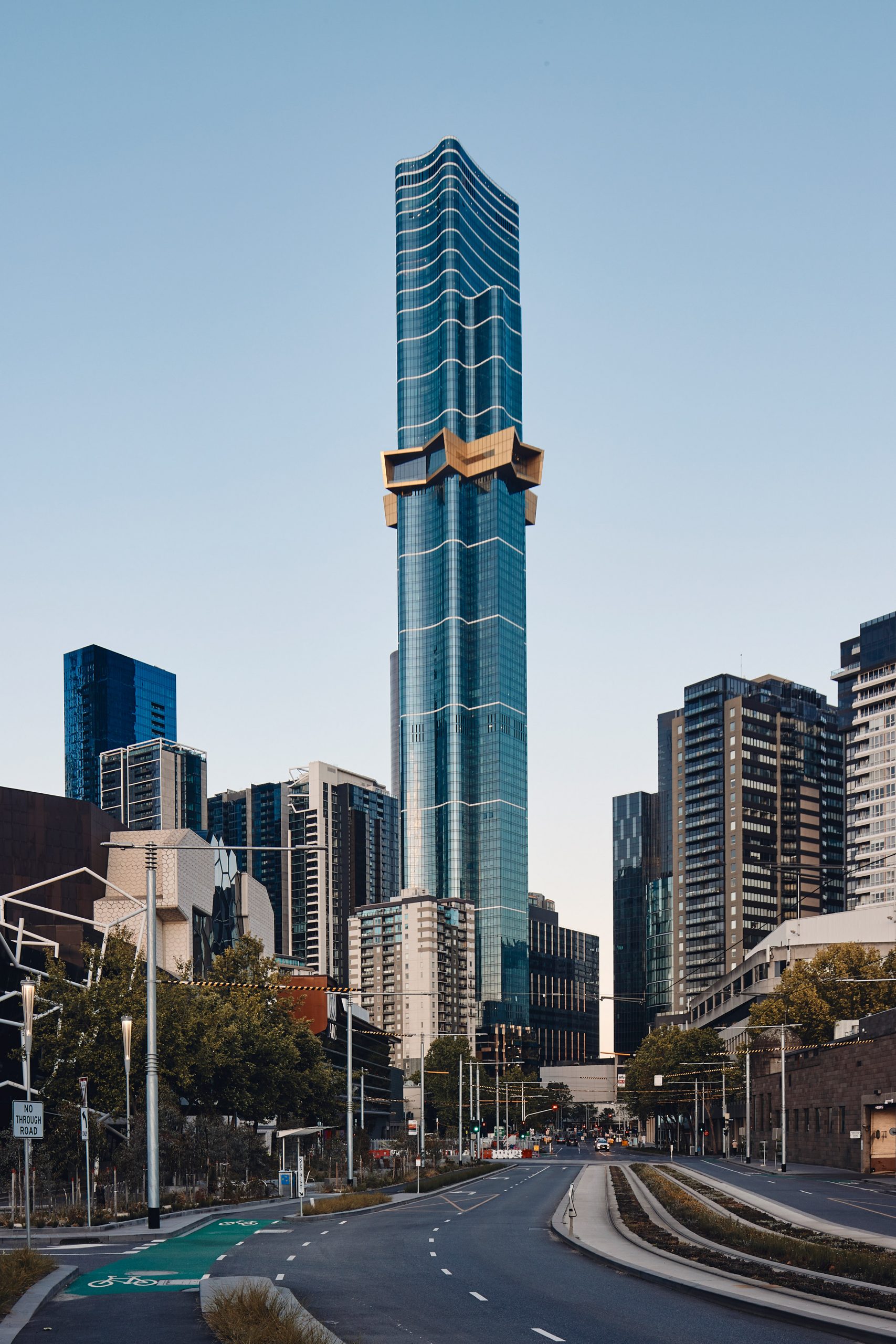This is a full-color photograph taken outdoors in a large city's downtown area during the daytime using natural light. The image is vertically rectangular, showcasing a clear sky with no clouds, which hints at the approaching sunset due to its lighter blue color. Dominating the center of the image is a striking blue skyscraper, approximately 50 stories high, with numerous windows that reflect a shiny, pastel blue hue. Notably, about two-thirds up this central building are distinctive golden triangular sections, giving it a unique and eye-catching appearance.

The photograph features a bustling urban street scene at the bottom. It depicts a busy four-lane road, with a median that appears to have been recently dug up to plant flowers and trees. Alongside the road, there's a walkway, various traffic signs including one indicating "No Through Traffic," and numerous streetlights dotting the scene. Some trees and clusters of people are visible as they navigate the city's streets, adding to the lively atmosphere. In the distance, more skyscrapers fill the skyline, further emphasizing the urban setting. This detailed composition highlights the grandiosity of the centerpiece skyscraper and the dynamic environment of the city.